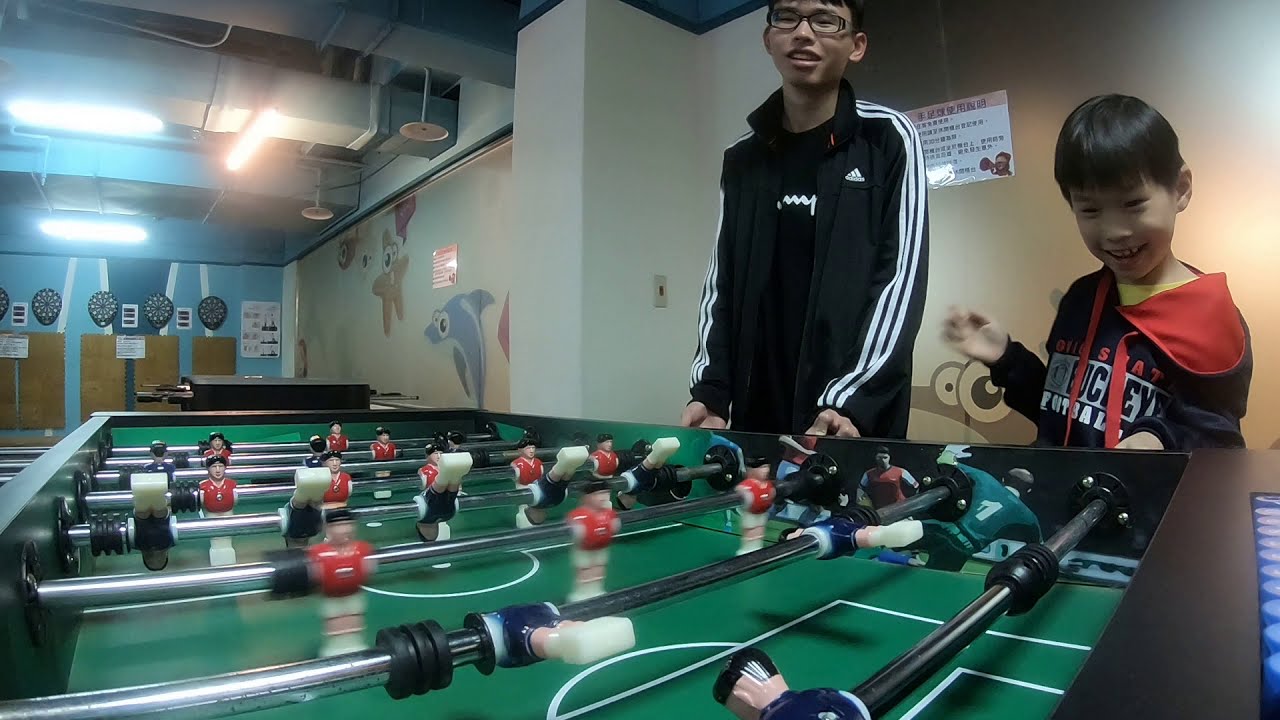The image is a detailed, color, landscape-oriented photograph capturing a vibrant moment inside a recreational center. Dominating the foreground is a foosball table, featuring a green playing surface with wooden figurines in different colors to represent the two soccer teams. The table's bars extend across its width, essential for maneuvering the players.

On the far side of the table are two young Asian boys engrossed in their foosball game. The boy on the right, approximately eight years old, is smiling and spinning the foosball sticks energetically to make the players move. He has short, straight black hair and wears a dark blue hooded sweatshirt with a red lining and some unreadable white and red graphics on the front.

Standing next to him on the left is an older boy, around 14 years old, who is about twice his height. He has short black hair and wears glasses. He is dressed in a black sports jacket with three white pinstripes running down the sleeves over a black Champion t-shirt.

The setting reveals itself as a recreational center through various background details. The white concrete walls are adorned with cartoonish aquatic characters, including dolphins, starfish, and goldfish. On the far left of the image, dartboards are mounted on the wall. There is also a sign with Asian writing behind the boys, reinforcing the cultural context of the environment. Overhead, the room is well-lit, further enhancing the cheerful atmosphere of this lively snapshot.